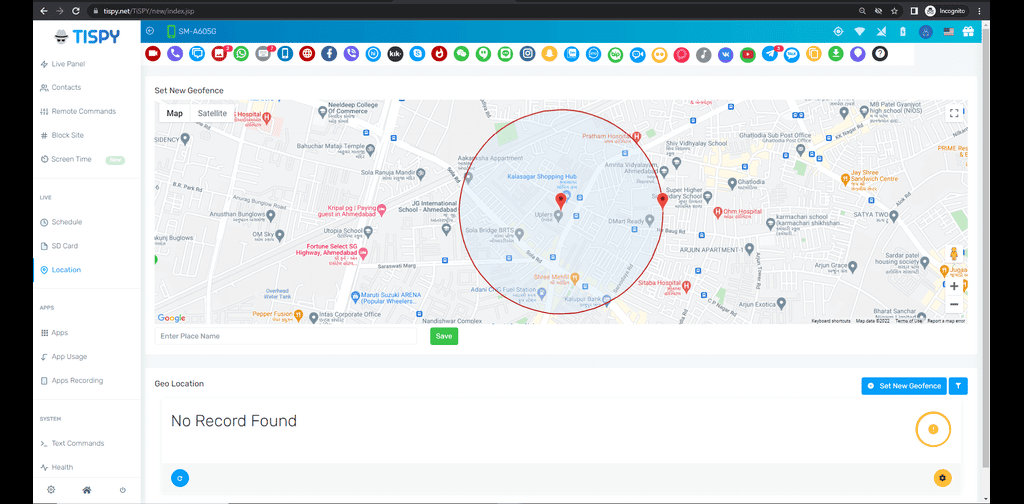Here is a refined and detailed caption for the image:

---

Screenshot of the "Tipsy" website interface. The website address, displayed in the browser's address bar, is "tipsy.nettsp/new/index.jsp". The browser window shows standard navigation buttons for back, forward, and refresh, along with an incognito mode indicator at the top right.

The website's layout features a vertical black border on both sides. On the left-hand side, a gray image of a figure wearing a detective-like hat accompanies the title "Tipsy". Below this, there is a navigation panel with the following options listed vertically: "Live Panel", "Contacts", "Remote Commands", "Block Site", "Screen Time", "Live Schedule", "SD Card Location", "Apps", "Apps Usage and Apps Recording", "System", "Text Commands", and "Health".

On the right-hand side, a blue bar at the top displays "SMA605G", likely indicating the phone's model designation. Beneath this bar, colorful icons are arranged next to a map interface that prompts the user to "Set New Geofence". The map section also includes fields for entering and saving a place name, though it currently shows "Geolocation: No record found".

---

This caption provides a clear, detailed description of the screenshot, highlighting the key elements and their layout on the interface.